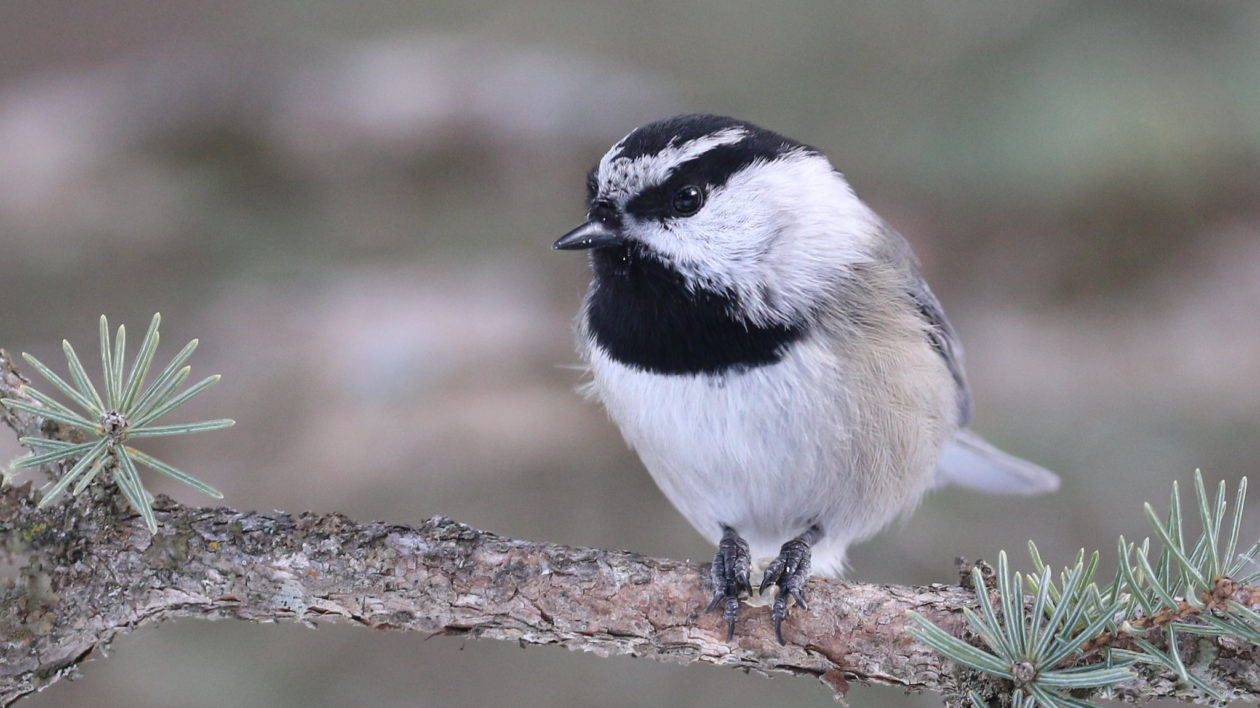A detailed, realistic horizontal photograph captures a small, fluffy bird resembling a Chickadee perched on a pine tree branch adorned with green pine needles. The bird has a distinct black cap on its head, a white belly, and light brown plumage towards its wings. Notably, it sports two black stripes extending from its beak through its black beady eyes and wrapping around to the back of its head, alongside a black beard. The bird is depicted showing a front view of its body and a quarter profile of its head, facing slightly left. It stands on the branch with scaly, blackish-gray feet, each displaying three visible toes. The branch itself has chipping bark and spots of moss. The background is a blur of browns and dull greens, likely indicating a forest setting during cooler fall or early winter, enhancing the focus on the bird's fine details and the textured bark.